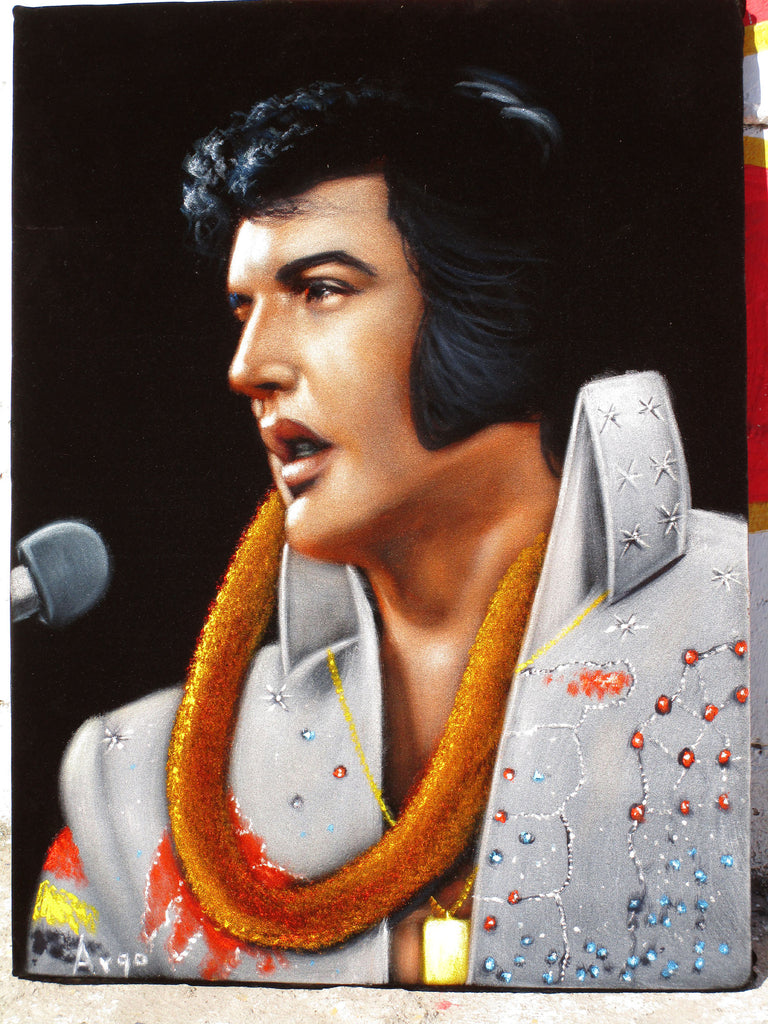The detailed image depicts Elvis Presley from the mid-chest up, set against a predominantly black background with subtle hints of red, yellow, and white on the right edge. Elvis is facing toward the left side of the frame, holding a microphone in his left hand, with his lips slightly parted as if he is singing. He has slicked-back black hair styled in a quintessential 70s fashion, with long sideburns extending to his chin.

Elvis is dressed in a striking white jumpsuit adorned with intricate blue and orange beading, and the outfit features a high, elaborately decorated collar with white star motifs. Adding to his iconic look, he wears a distinct orange, fuzzy lei around his neck, contrasting against the sparkly elements of his attire. A gold chain necklace with a dog tag can also be seen around his neck, which glistens against the textured surface of what appears to be a felt or velvet painting. In the lower left corner of the image, the signature "Argo" is visible, marking the artist's name. The image is vertical, approximately six inches tall and four inches wide, capturing the essence of Elvis in a moment of musical performance with a serious expression.